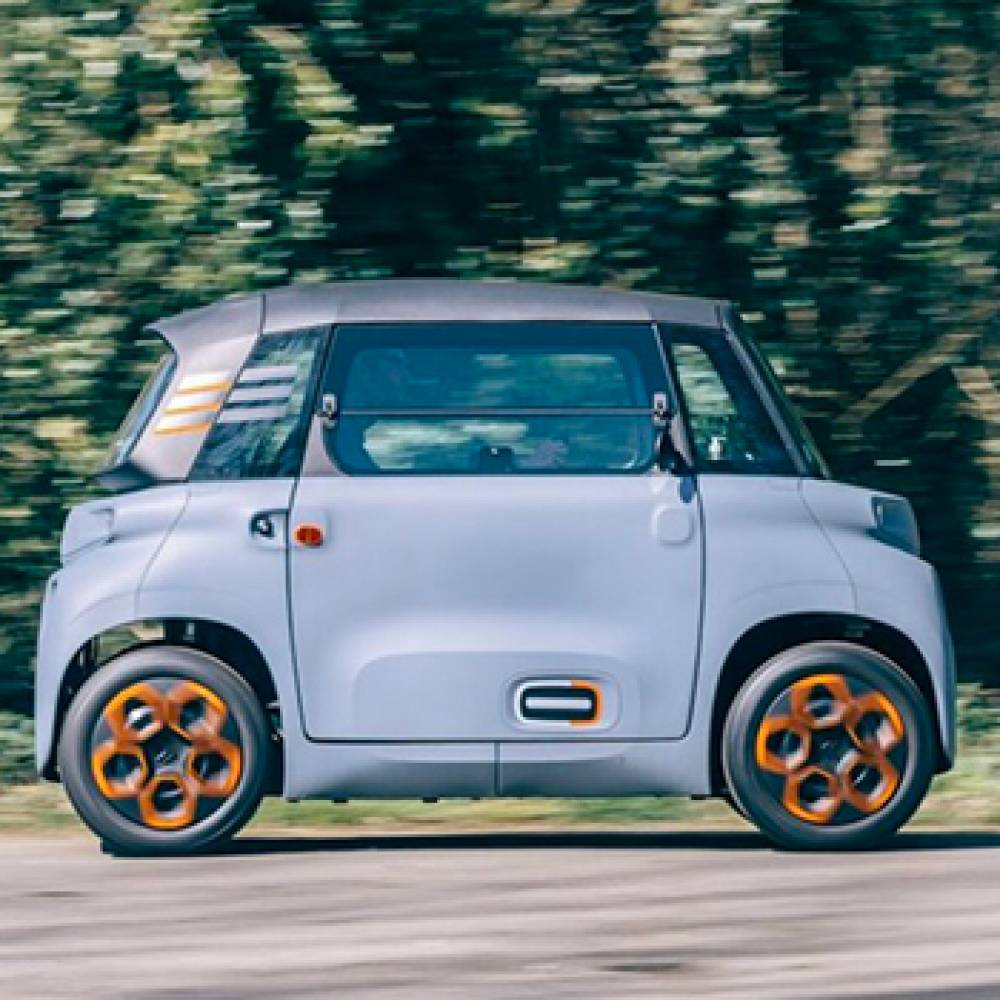The image features a compact, unusual European car, possibly electric, captured in motion against a blurred backdrop of trees on a sandy road. The car's design is boxy and stubby, akin to a golf cart or a smart city car, emphasizing functionality over sportiness. It is extremely tiny, with only one door and a front windshield that has a slight slope. The car’s body is a grayish-blue, and it sits low to the ground on black rubber tires. The wheels are adorned with distinctive orange pentagon-shaped designs, five on each, and the door handle is orange as well. The scene has a color palette dominated by greens, grays, browns, and the striking oranges on the wheels. From the side view provided in the image, the car is facing to the right.